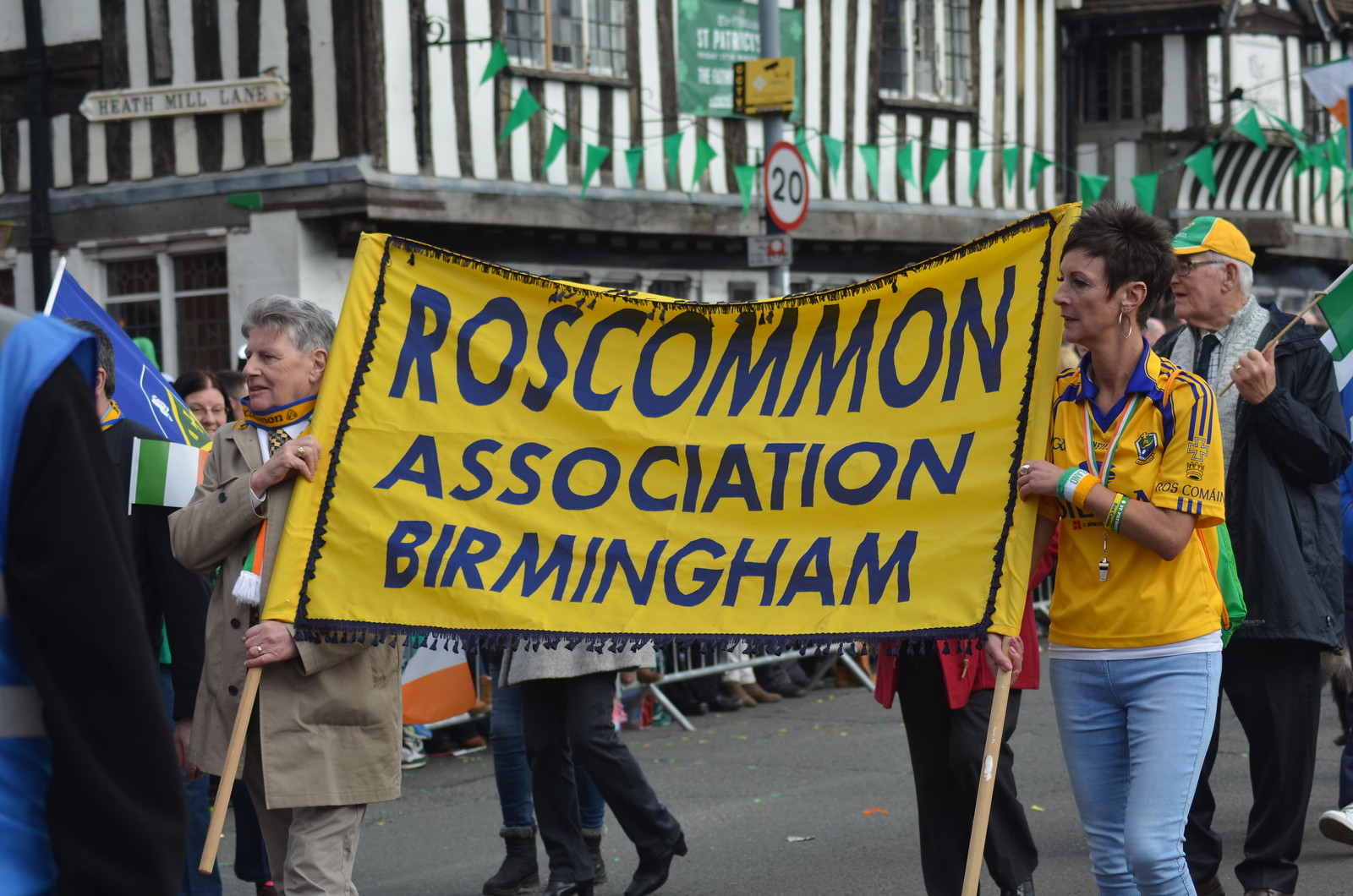A lively street scene captures two individuals holding a striking yellow banner bordered with a blue square that reads “Roscommon Association, Birmingham” in blue text. The woman on the right, identifiable by her short black hair, wears a yellow jersey with blue stripes along the arms and collar, paired with light blue pants. A distinctive wristband featuring yellow, white, and green sections adorns her arm. On the left, an elderly man with short gray and white hair is dressed in a light gray or tan jacket and khaki pants, his gold rings visible as he grips the banner’s wooden poles. Surrounding them, a festive parade atmosphere is suggested by additional participants and observers, some waving flags with green, white, and orange stripes. The backdrop includes a distinctive building with a second-floor wall patterned in alternating white and black stripes, accompanied by a gray pole with a 20 mph speed limit sign. Above the scene, a banner festooned with green triangles adds to the celebratory vibe.